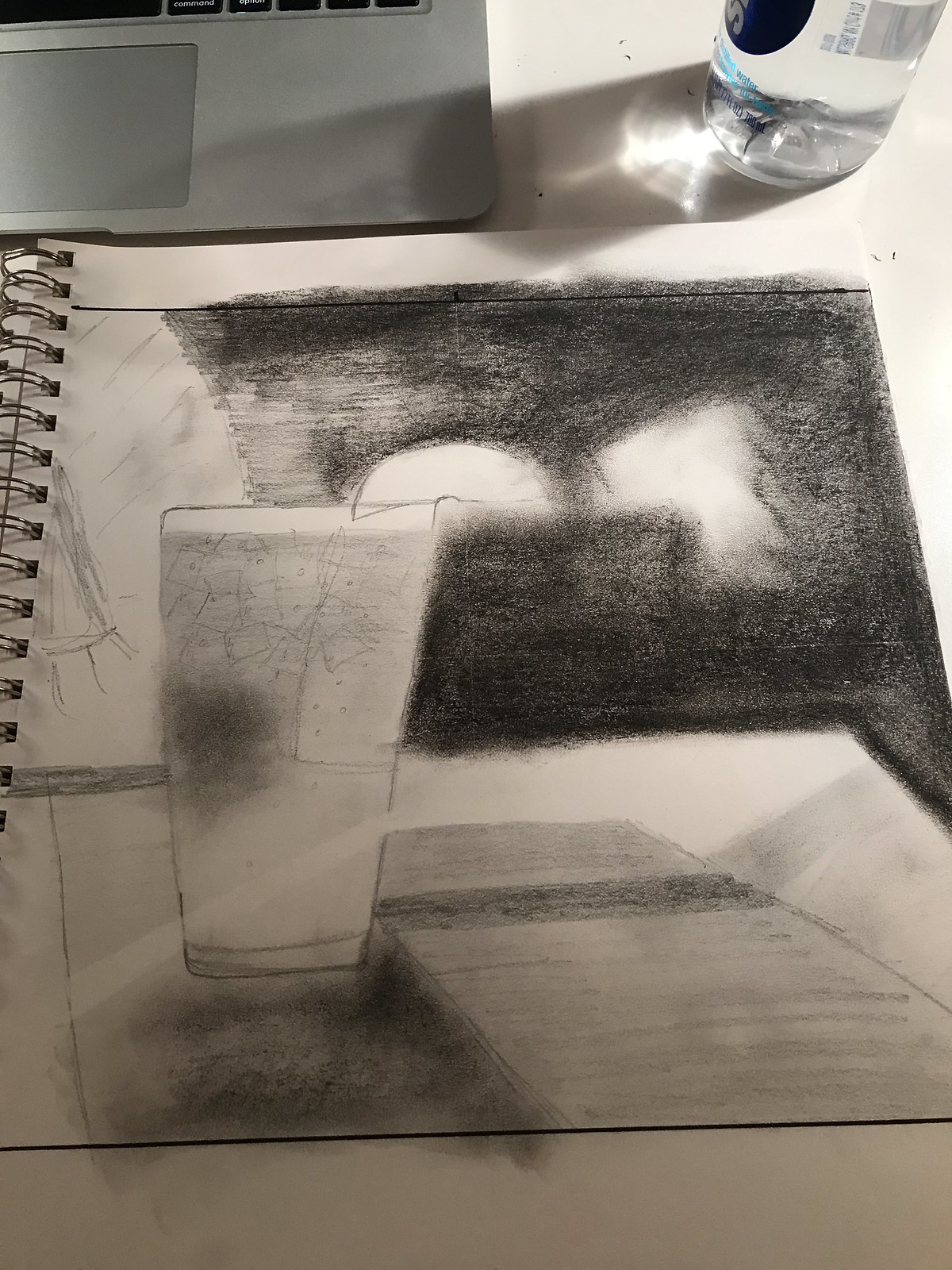A detailed sketch in a white spiral-bound notebook captures a tall glass that could be holding a pint of beer or lemonade. The glass features a foamy head, suggesting it contains a frothy beverage. Adjacent to the glass, there's a piece of paper or a book marked with graphite strokes, evoking the idea of writing. The scene is set on a table, backed by the corner of a wall, creating a distinct right angle. The background is predominantly dark, interrupted by two white shapes. One arch-shaped form, likely representing a slice of lemon, rests on the rim of the glass. The other irregularly shaped white blob remains ambiguous, seemingly part of the background wall.